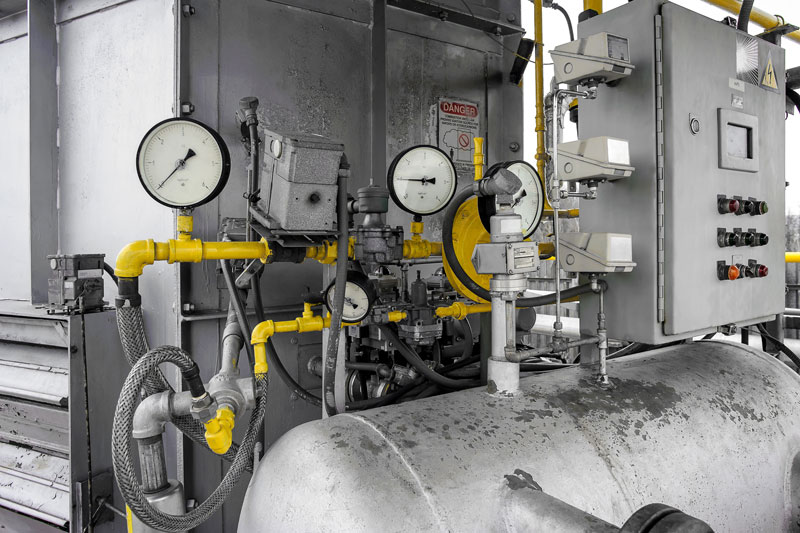This color photograph captures an array of industrial equipment, prominently featuring a large tank in the foreground. The tank, characterized by its gray metal hue, is outfitted with bright yellow tubes extending outward. Accompanying these tubes are numerous instruments equipped with prominent dials, presumably for measuring pressure or other critical parameters. Behind the tank sits a small-room-sized metal structure of similar gray coloration. Attached to this structure is a noticeable sign marked with the word "Danger" in white text set against a red background, accompanied by a red circle with a horizontal line through it, warning against certain actions. Adjacent to the tank on the lower right, an oil drum is visible. The scene also showcases a variety of silver pipes, hoses, switches, and an electrical box. The setting appears to be outdoors, and the overall configuration of the machinery hints at its functional complexity, resembling a substation or similar mechanical installation.